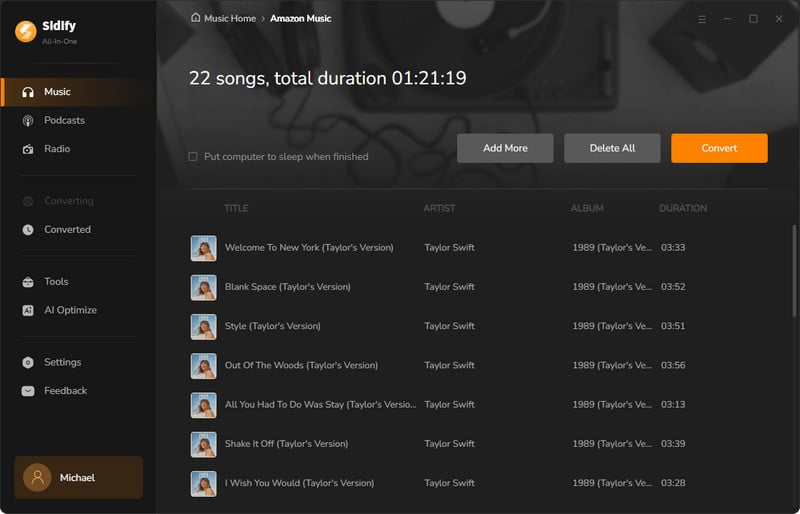**Detailed Caption for Screenshot from Amazon Music Web Player:**

This screenshot, taken from the Amazon Music web player on a monitor, features an overall gray background adorned with subtle shadow imagery. On the left-hand side, there is a prominent column. At the top of this column, near the right of an orange circle containing a white squiggly line, the bold black text reads "Sitify All in One."

Directly beneath this, an orange-marked area features an orange home button accompanied by the word "Home" in bold, also in orange. Below this, in a very light font against a light background, the text reads "Converting." Underneath that section, a gray clock icon appears with the word "Converted" beside it. At the bottom of this column is a toolcase icon labeled "Tools."

In the center of the screenshot, a bar at the top reads "Amazon Music Web Player." Below this bar, in bold black text, it states "10 songs, total duration 34 minutes and 46 seconds."

To the left, an option is visible saying "Put computer to sleep when finished." On the right side, there are three buttons; two are white with black text reading "Add More" and "Delete All." The third button is orange with white text that says "Convert."

Below these buttons, four labels are present: "Title," "Artist," "Album," and "Duration." To the far left, there's a square pink icon that is blurry and illegible.

The list of songs includes:
1. "I Forgot That You Existed"
2. "Cruel Summer"
3. "Lover"
4. "The Man"
5. "The Archer"
6. "I Think He Knows"
7. "Miss Americana & The Heartbreak Prince"

Under the "Artist" column, each song is attributed to "Taylor Swift." The "Album" column lists "Lover" for all tracks, and the "Duration" column provides minute timestamps for each song.